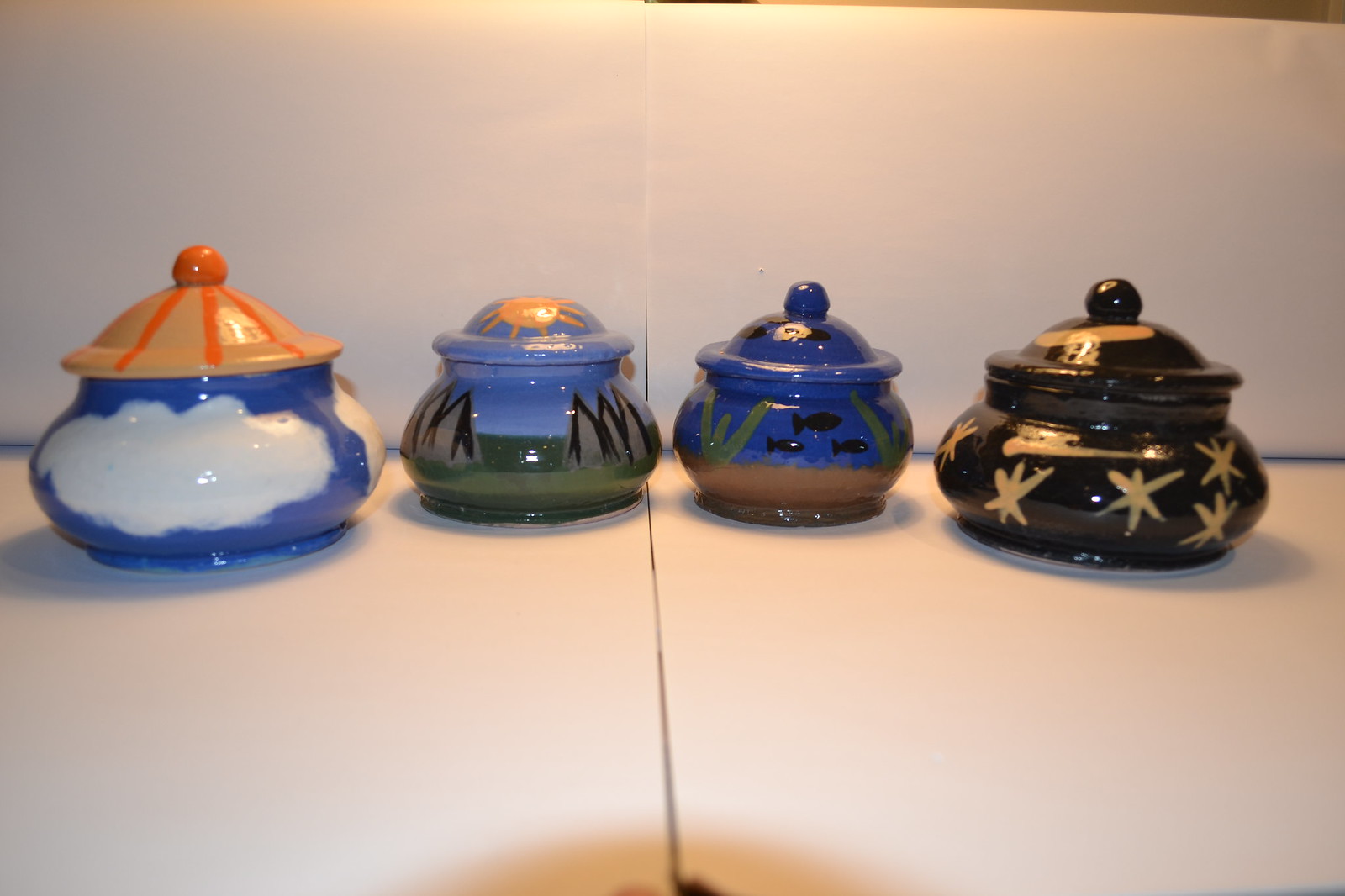This photo, taken indoors, showcases four handcrafted ceramic jars arranged on a pristine white countertop against a white backdrop. Each jar is uniquely painted, reflecting diverse themes and artistic detail. 

Starting from the left, the first jar is the largest and features a serene blue sky with a large white cloud, its lid adorned with a peach hue, topped with a dark orange knob from which three orange stripes emanate. To its right sits a smaller jar illustrating a picturesque underwater scene. This jar transitions from sandy brown at the base to bright blue water, populated with green aquatic plants, gray rocks, and black fish. Its lid is blue, crowned with an orange sun.

The third jar, artistically, presents a terrestrial landscape, displaying vibrant green terrain beneath a sky-blue section, reminiscent of a scene where the land meets the sky. The jar’s lid continues the aquatic theme, painted blue with three black fish circling the top.

The final jar on the right is slightly larger and cloaked entirely in black. It is adorned with gold stars, creating a celestial landscape. The lid mirrors the jar's color with an intricate golden design, topped by a matching black knob.

The base's subtle black line running down the center of the countertop adds a hint of division, emphasizing the curated placement of these charming jars, making them appear almost like treasured artifacts in a minimalistic space.